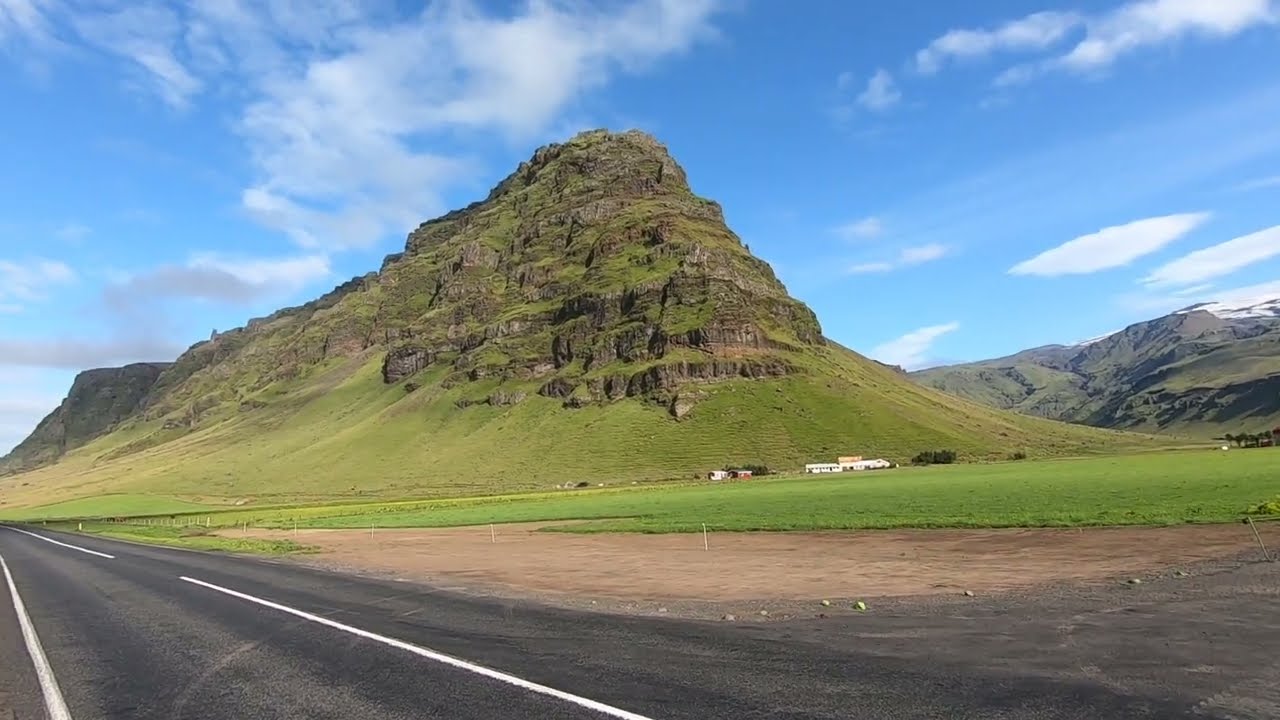An expansive outdoor scene captures a majestic, towering rock formation, likely reminiscent of those in the Rocky Mountains or Utah. The formation, which seems to be hundreds of feet tall, is characterized by green grass and moss, along with sheer cliff ledges where pieces have fallen off. Above, a mostly blue sky is dotted with some white and gray clouds, indicating a sunny day. The image, taken during the daytime, shows the light illuminating the rock formation from the side.

In the foreground, there is a black asphalt road with white traffic lines, possibly a highway, running parallel to the scene. A dirt pathway borders this road, leading into a wide grassy field that spans much of the area. This field gradually transitions into more rugged mountainous terrain, with additional snow-capped peaks visible in the distance to the right.

Off in the far distance beneath the peaks, a housing complex with white buildings can be seen, along with a few scattered trees. The road includes a parking strip and appears to be a single lane in each direction. There are no visible signs or text in the image, further emphasizing the untouched, natural beauty of the landscape. The vibrant colors of the scene range from various shades of green, brown, and tan to the crisp whites and blues of the sky and clouds.